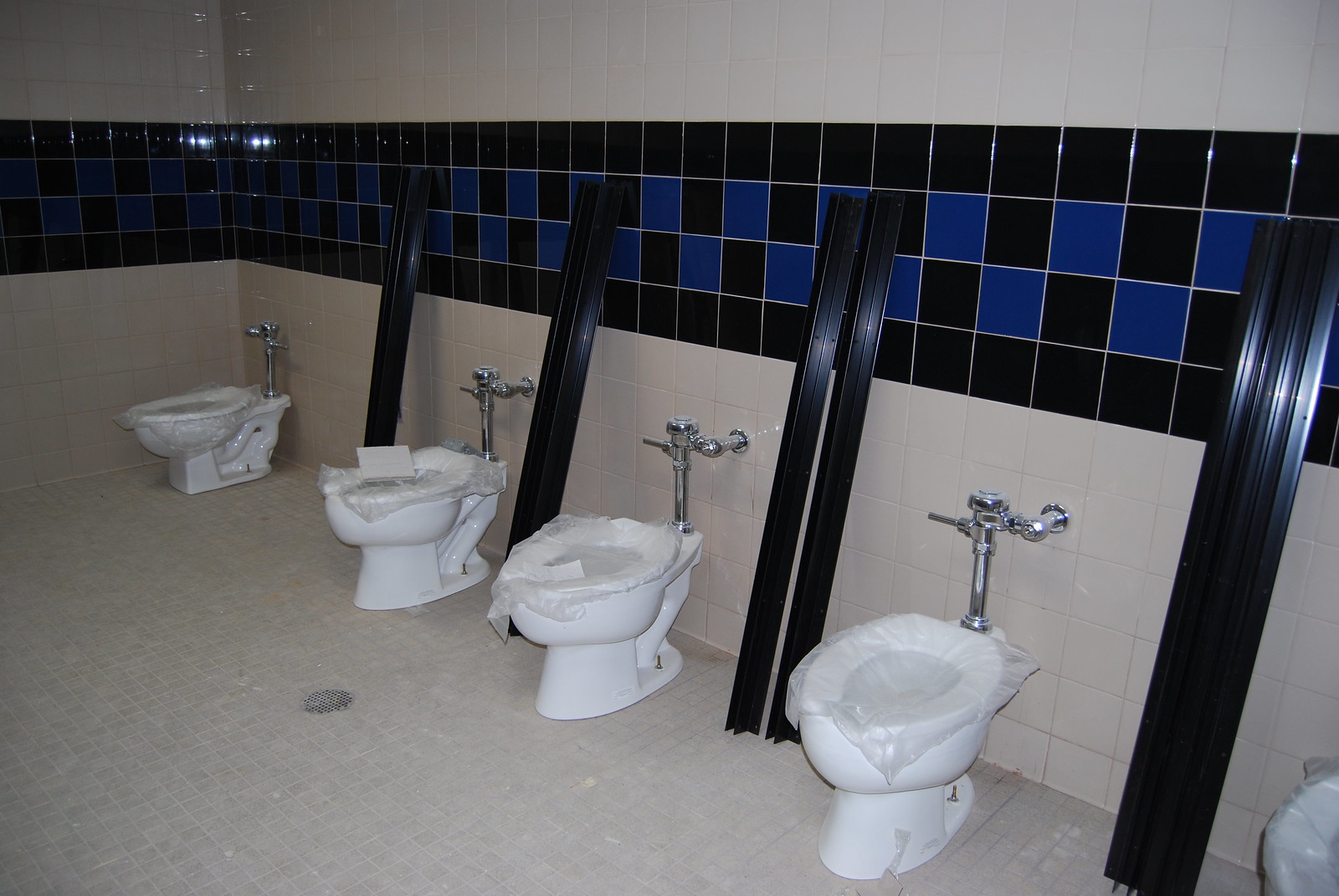The image captures a public restroom currently under construction, featuring five wall-mounted, white porcelain toilets, each without individual stalls. The toilets are uniformly covered in protective plastic, signaling ongoing installation. The restroom has a white tiled wall with a striking central band of alternating black and royal blue tiles. The floor is also tiled, distinguished by a central drain, indicative of an efficient drainage system. Notably, the toilet farthest from the photographer is spaced at roughly twice the distance from its neighbor compared to the spacing between the other four, suggesting a future handicapped-accessible stall. Leaning diagonally against the wall are black slats or potentially dividers, hinting at the future installation of stall separators to ensure privacy. The restroom's unfinished state is underscored by the visible metal piping and flushing mechanisms, as well as the absence of lids on the toilets.